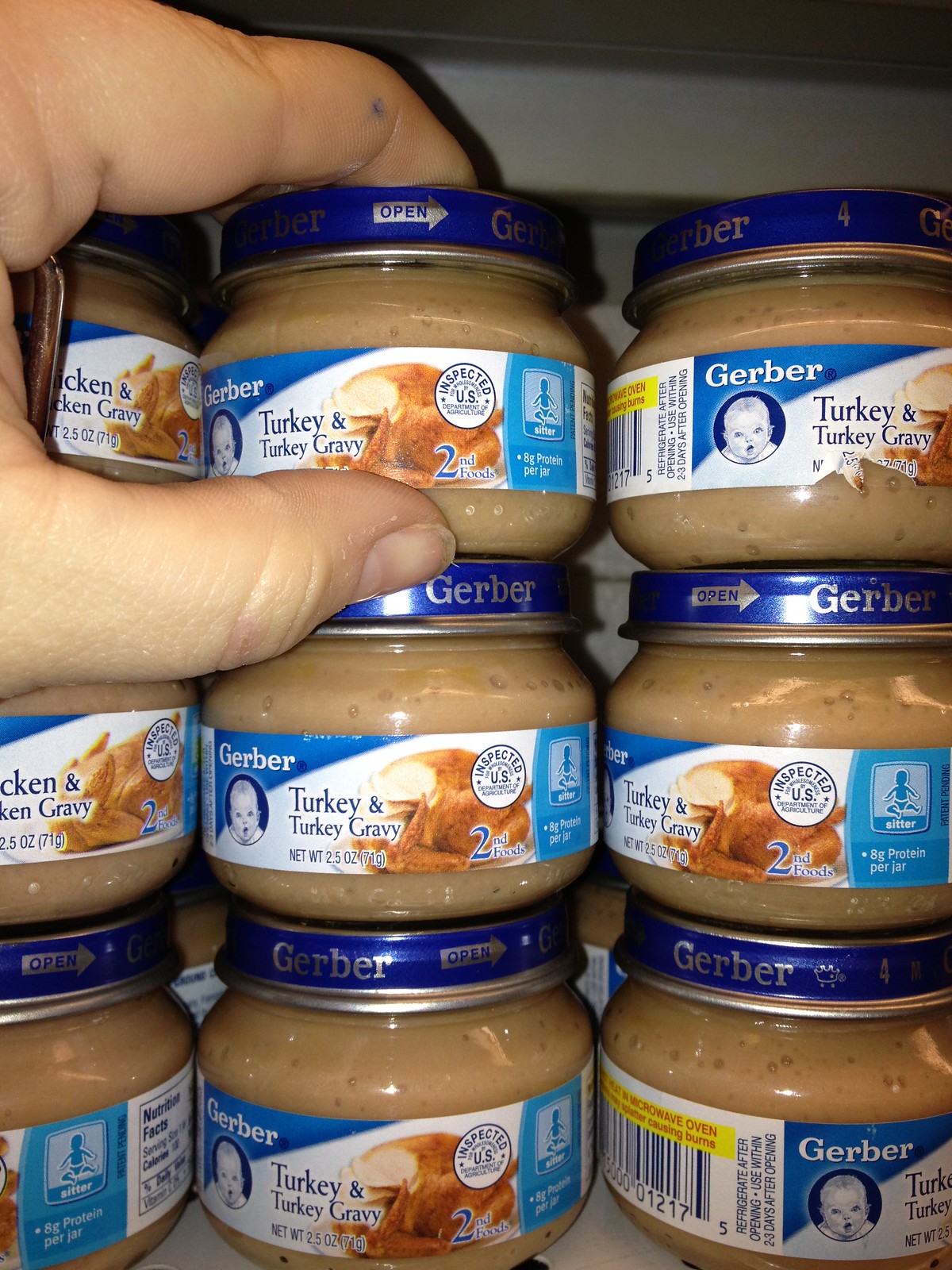The image features nine cans of Gerber baby food, each weighing 2.5 ounces (71 grams), neatly arranged in three stacks of three on a shelf. The specific flavor is Gerber Turkey and Turkey Gravy. A person's left hand is partially visible in the frame, with their thumb and index finger grasping a jar from the middle stack. The context of the setting—whether it's a home pantry or a store shelf—remains ambiguous.